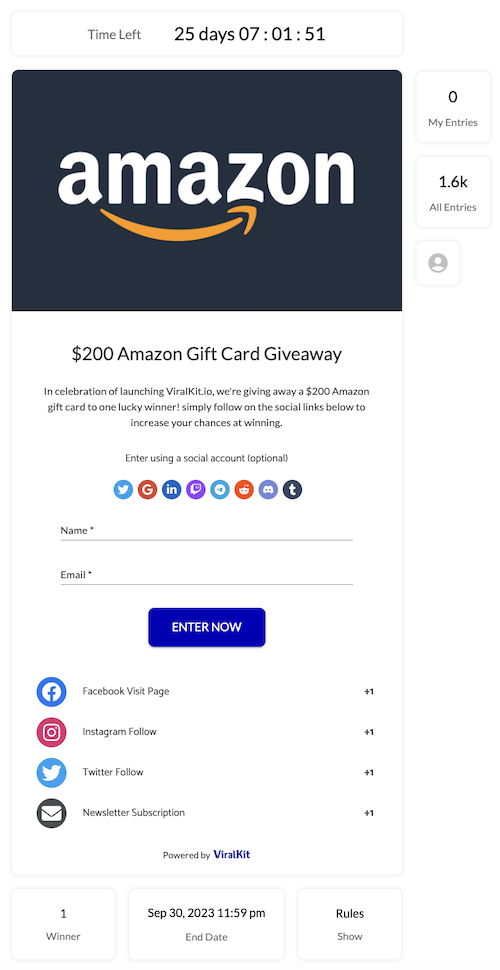Here is a cleaned-up and detailed caption for the described image:

---

The screenshot depicts a promotional offer on a cell phone. At the top, a grey-outlined rectangle in black lettering displays a countdown timer reading "Time Left: 25 days, 07:01:51." Below this, there is a prominent black square featuring the word "Amazon" in bold white letters, with an arrow pointing from the letter "A" to the letter "Z" beneath it. The text "Amazon $200 Gift Card Giveaway" follows in black letters. The partially visible text below reads "In celebration," but the remaining words are too small to discern. The instructions "Enter by using social media account" are followed by a series of social media icons, including Twitter, TikTok, a red circle with a "G," a blue circle with "IN," a purple circle, and another blue circle with a white design inside. The form fields for "Name" and "Email" appear next, each with black text and grey lines for input. Beneath these fields is a purple button labeled "Enter Now." The entry form concludes with options to follow or subscribe: "Facebook Page," "Instagram Follow," "Twitter Follow," and "Newsletter Subscription."

---